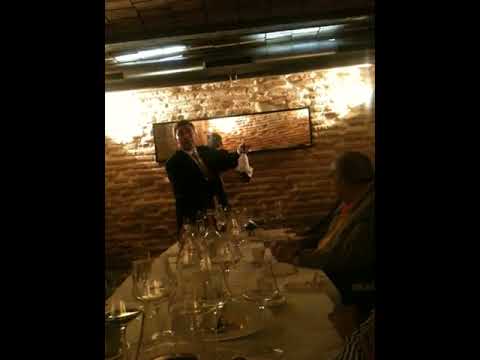This is a dimly lit, full-color, rectangular photograph taken indoors, possibly in a restaurant that gives off a subterranean, cavernous vibe. The picture is centered and framed with thick black borders on both the left and right sides. At the focal point is a long table covered with a white tablecloth, set with numerous glass carafes and containers. The table is populated with a couple of guests. On the right side of the table sits a large, heavyset man with gray hair, seemingly of Caucasian descent, intently observing a man at the head of the table. 

This man, standing at the end of the table, wears a black suit with a tie and a white shirt beneath. He holds something white in his hand, speculated to be a small bell or potentially a wine bottle, as he appears to be making a speech or toast. Behind him, the backdrop consists of a red brick wall adorned with what looks like a mirror or a rectangular sign that possibly reflects more brick wall. The setting gives an impression of being in a private dining space, accentuated by subtle sconce lighting above, adding to the photograph's intimate ambiance.